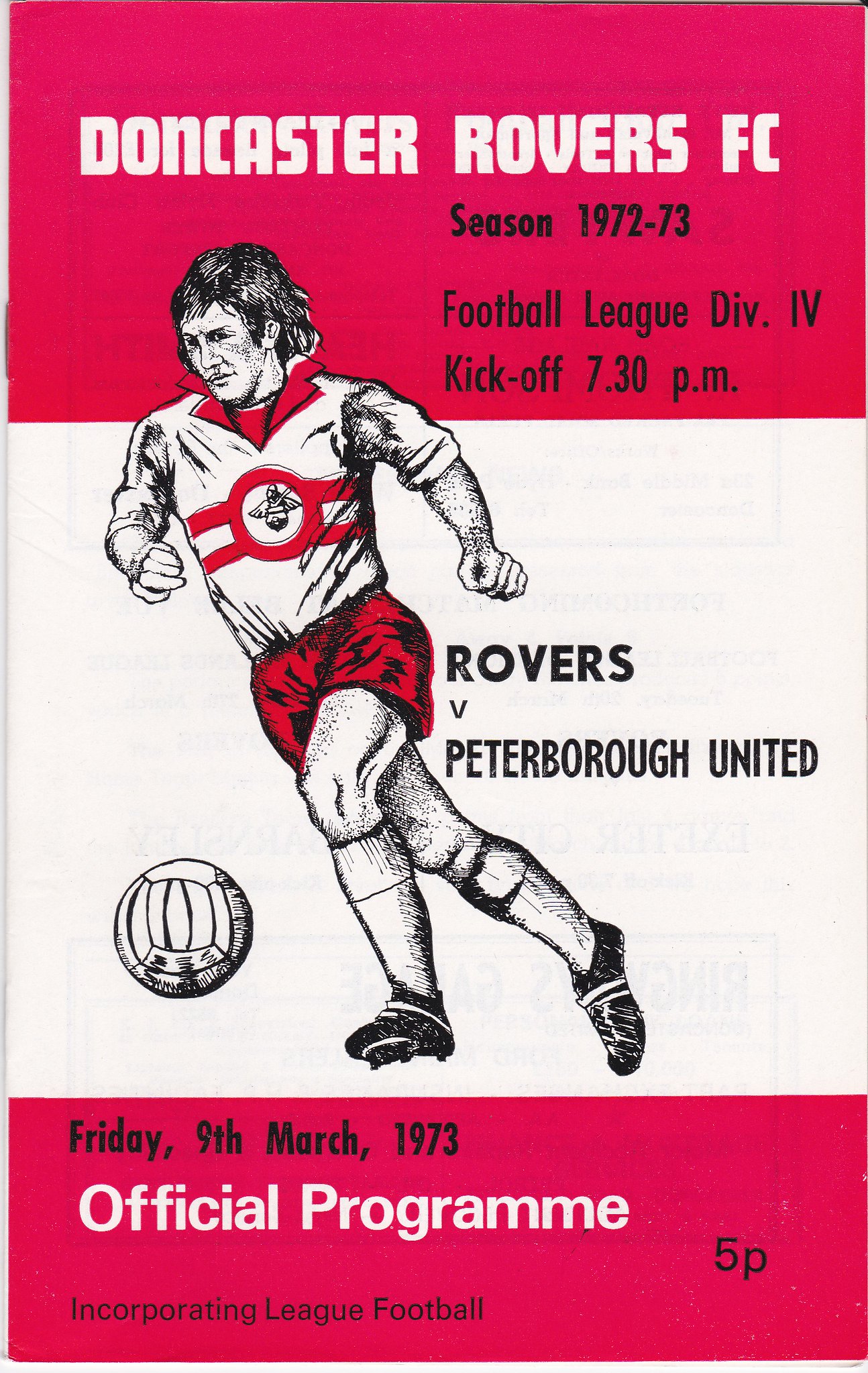The front cover of the official program for Doncaster Rovers FC's match against Peterborough United on Friday, 9th March 1973, prominently features the team's iconic red and white colors. The top portion of the cover, with its red background, displays "Doncaster Rovers F.C." in white lettering, followed by "Season 1972-73" and "Football League Division 4" in black text, along with the kickoff time of 7:30 p.m. The center section, set against a white background, showcases a detailed graphic artist's drawing of a football player with long hair, dressed in red shorts, knee-high socks, and a white jersey with a red collar and logo. He is seen running and kicking a soccer ball. Adjacent to the drawing, the matchup "Rovers vs. Peterborough United" is printed in black text. The bottom portion of the cover, also with a red background, includes the date, "Friday, 9th March 1973," and additional details like "Official Program" and "Incorporating League Football," with a price indication of "5P."